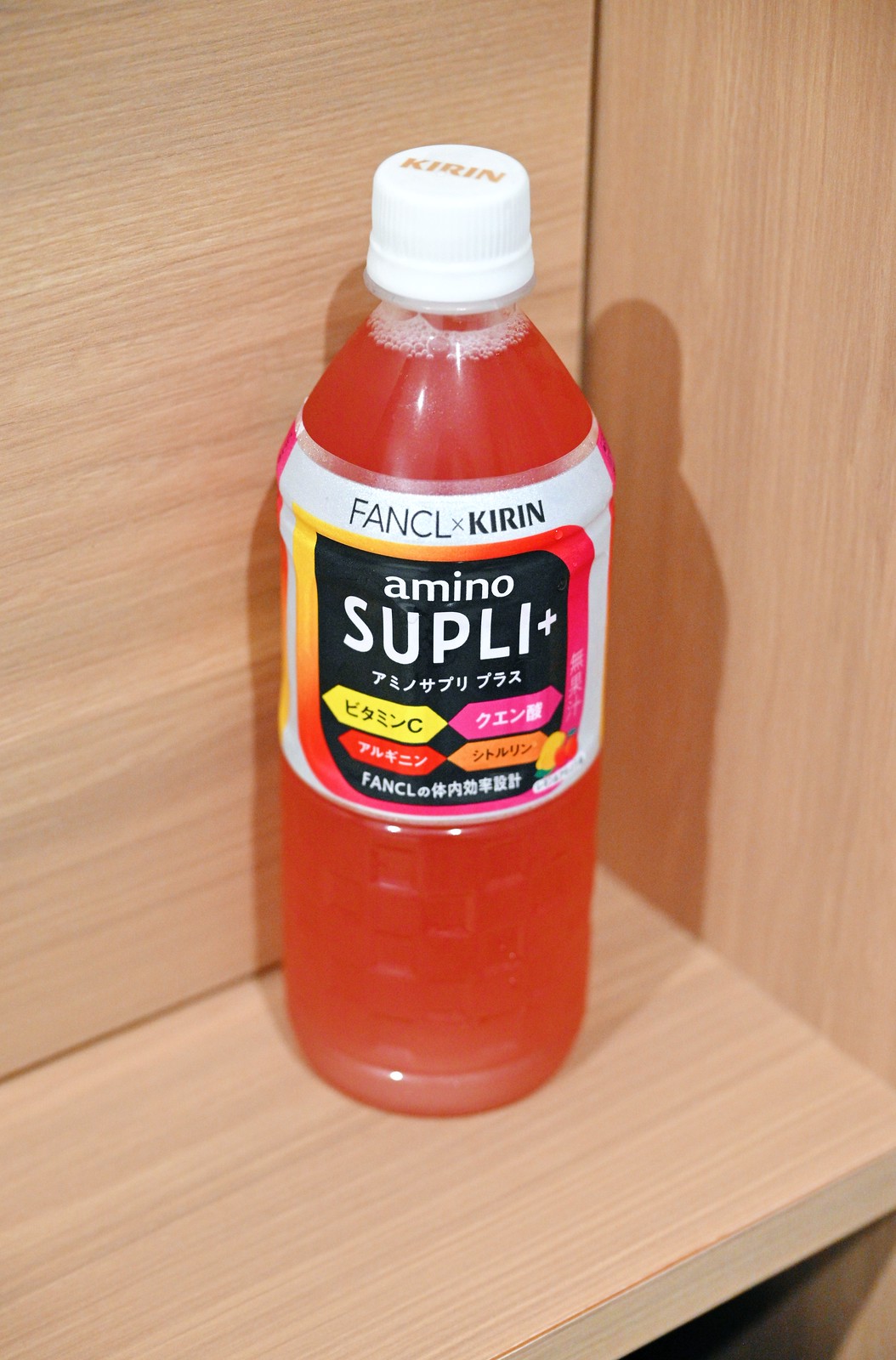This photograph showcases a clear plastic bottle, approximately six inches tall, resting on a light, natural wooden shelf within a wooden cabinet. The bottle is filled to the top with a reddish-orange liquid and is sealed with a white plastic cap featuring red text. The label on the bottle prominently displays "F-A-N-C-L x K-I-R-I-N" in black lettering at the top, followed by "Amino S-U-P-L-I" in bold white letters against a black background with surrounding orange and pink lines. Below this, there is Chinese calligraphy written on variously colored rectangles in shades of yellow, pink, red, and orange. The setting of the bottle, in a brown, cube-type shelf, contributes to the image's warm, natural ambiance.